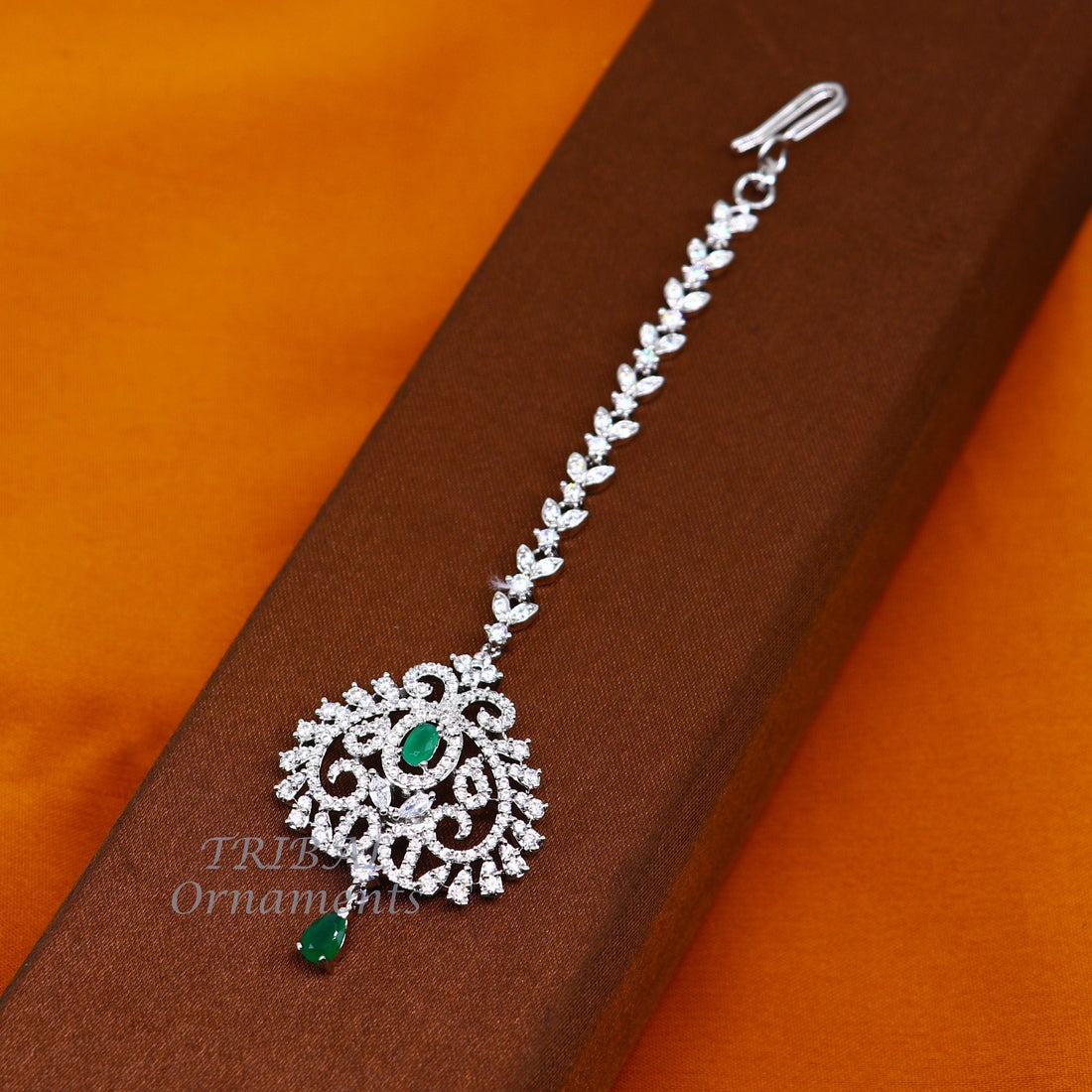The image showcases a professional photograph of an intricately designed piece of jewelry, possibly a pendant or a brooch, resting on a reddish-brown rectangular box set against a vivid orange fabric. The jewelry itself is predominantly silver, featuring a detailed floral design running along its chain and main structure. The pendant boasts sparkling white gemstones or diamonds arranged in a scrolling pattern, with a striking oval-shaped green emerald at its center and another emerald hanging beneath it. The piece also has rows of leaf-like designs, each adorned with tiny diamonds or gems, adding to its elaborate craftsmanship. The text "tribal ornaments" can be partially seen beneath the jewelry, adding a hint of context to its cultural inspiration.